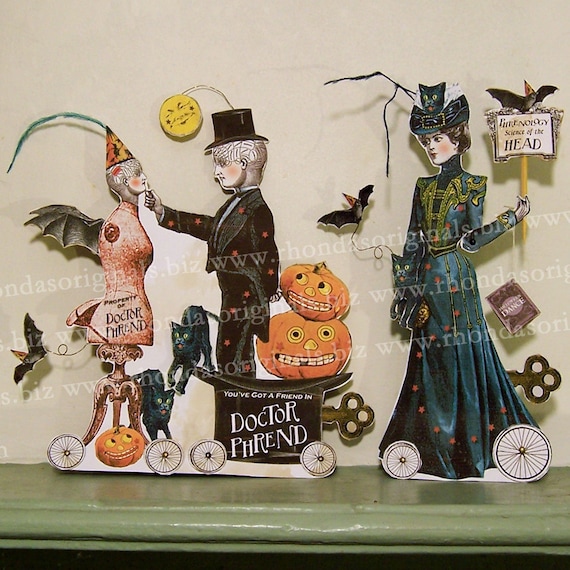The image depicts a whimsical Halloween scene featuring wind-up cardstock cutouts of three figurines. Centered is "Dr. Friend," spelled P-H-R-E-N-D, adorned in a black jacket and top hat, standing in a much larger top hat that bears the phrase "You've got a friend in Dr. Friend." Behind him, two pumpkins with silly faces are stacked, adding to the festive atmosphere. The doctor looks at a mannequin dressed in a creepy costume with bat wings and a party hat. Surrounding them are two black cats with playful expressions. 

To the right, a woman in a gothic blue dress holds a sign reading "Phrenology Science of the Head" and wears a distinctive hat decorated with ravens and a black cat sitting atop it. Her attire and the black stars scattered around the scene enhance the eerie, old-fashioned setting. A smiling moon, connected to Dr. Friend’s top hat by a wire, hovers above, adding a surreal touch to the peculiar, muted-colored tableau.